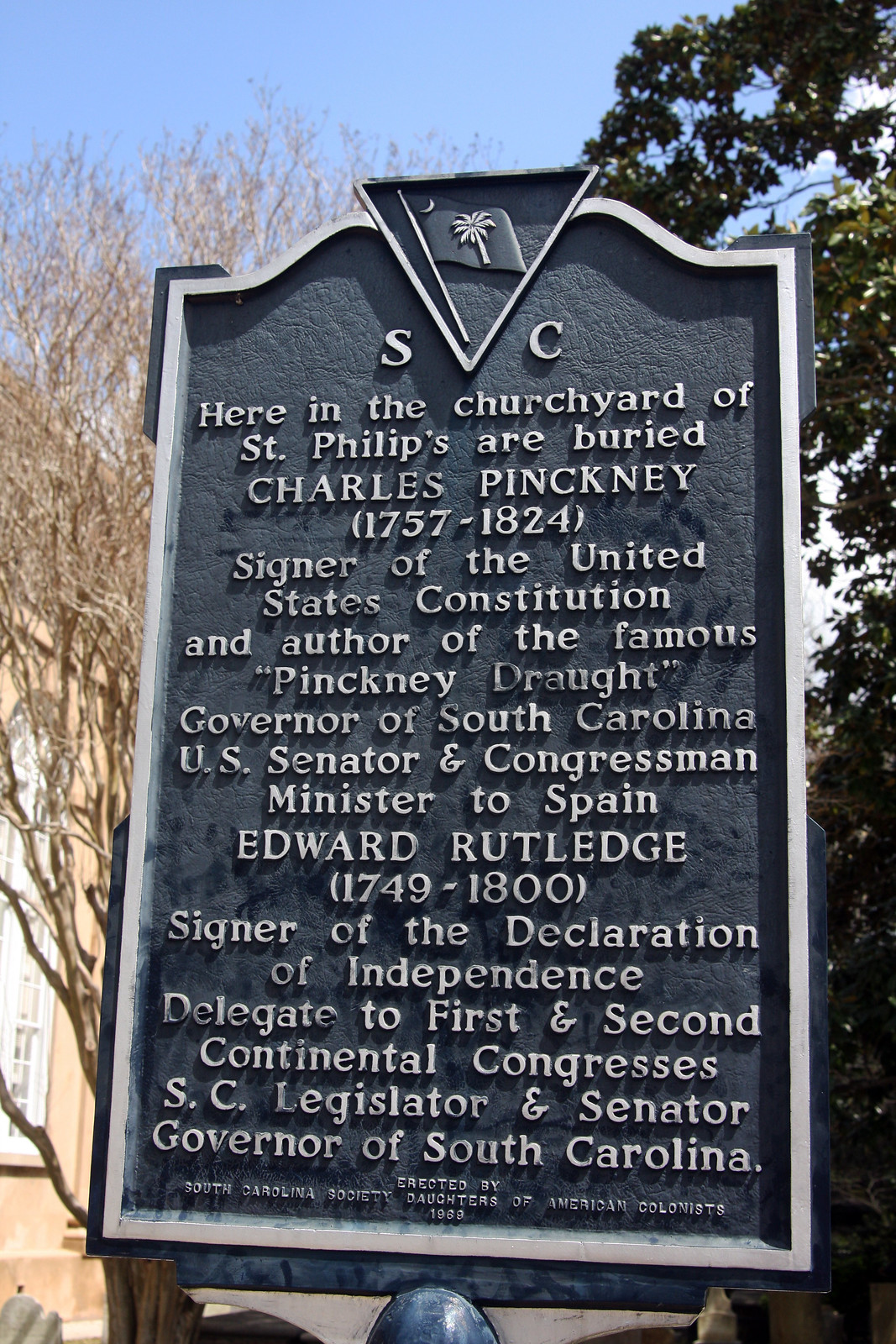This photograph captures a large, vertical, rectangular plaque with a bluish-gray background and white text and border situated at the center of the image. Prominently featured at the top of the plaque is an upside-down triangle containing a 2D depiction of the South Carolina flag: a white palmetto tree and crescent moon on a flagpole, alongside the letters 'SC' in the same white color. Below the triangle, the plaque reads, "Here in the churchyard of St. Phillips are buried Charles Pinckney, 1757 to 1824, signer of the United States Constitution and author of the famous Pinckney Draft, governor of South Carolina, U.S. senator and congressman, minister to Spain, and Edward Rutledge, 1749 to 1800, signer of the Declaration of Independence, delegate to the First and Second Continental Congresses, SC legislator and senator, and governor of South Carolina." The plaque also contains smaller, less legible text at the bottom, which mentions being erected by the South Carolina Society Daughters of American Colonists in 1969. The background features contrasting trees: a leafless, brown-branched tree to the left and a lush, green-leaved tree casting shadows to the right. Topping off the scene is a blue skyline peeking through the foliage.